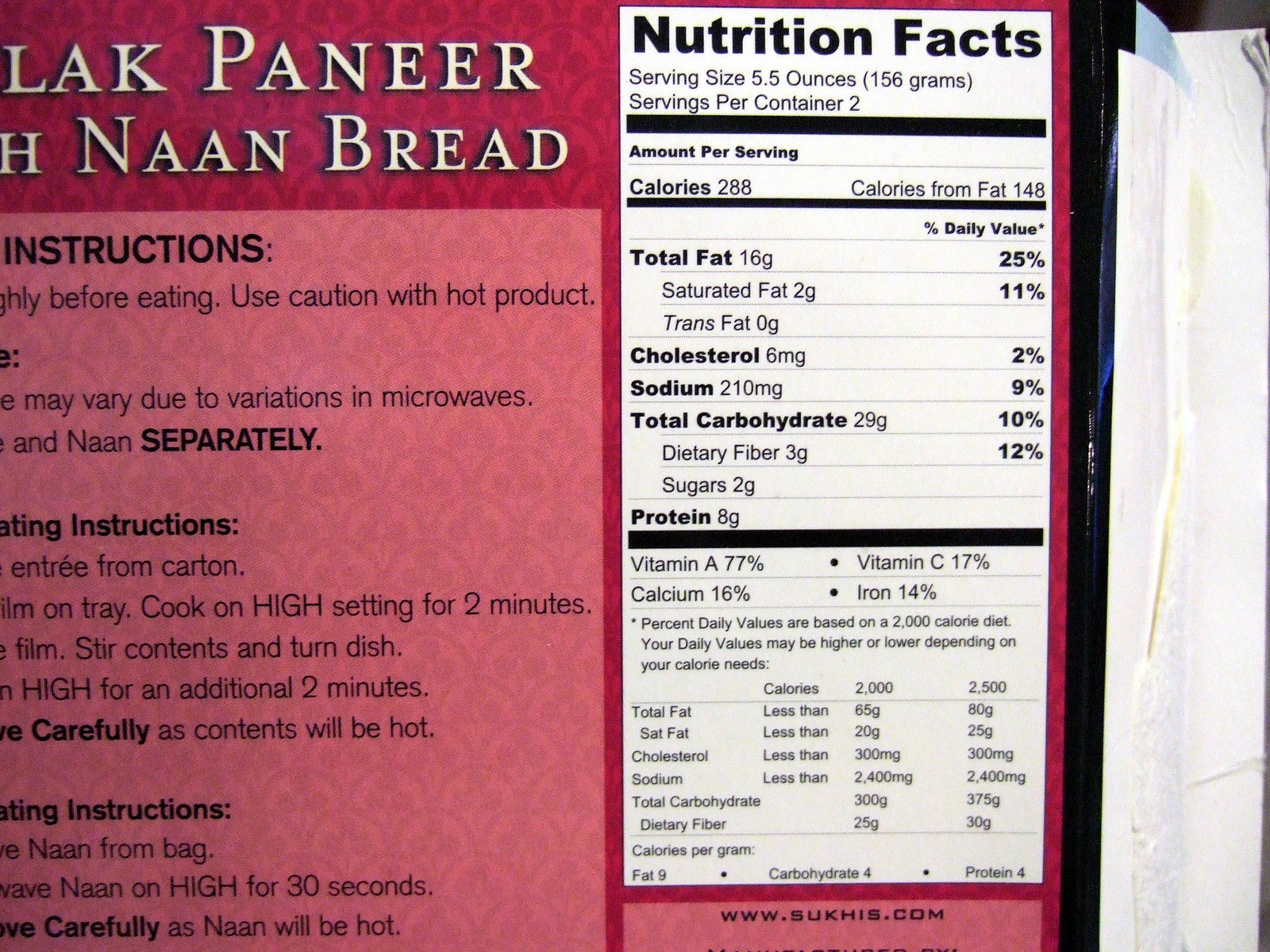This image shows the backside of a cardboard box for L.A.K. Pannier Naan Bread. The box, which has been opened, is predominantly printed in a vibrant pink color. The left side of the box features detailed heating instructions set within a pink rectangular section. These instructions include steps for removing the naan bread from the carton and cooking them individually, along with a cautionary note that the contents will be hot. On the right side, there is a white nutrition facts panel outlining the serving size, nutritional values, vitamins, and minerals contained in the bread. At the bottom of the box, the website www.succus.com is prominently displayed.